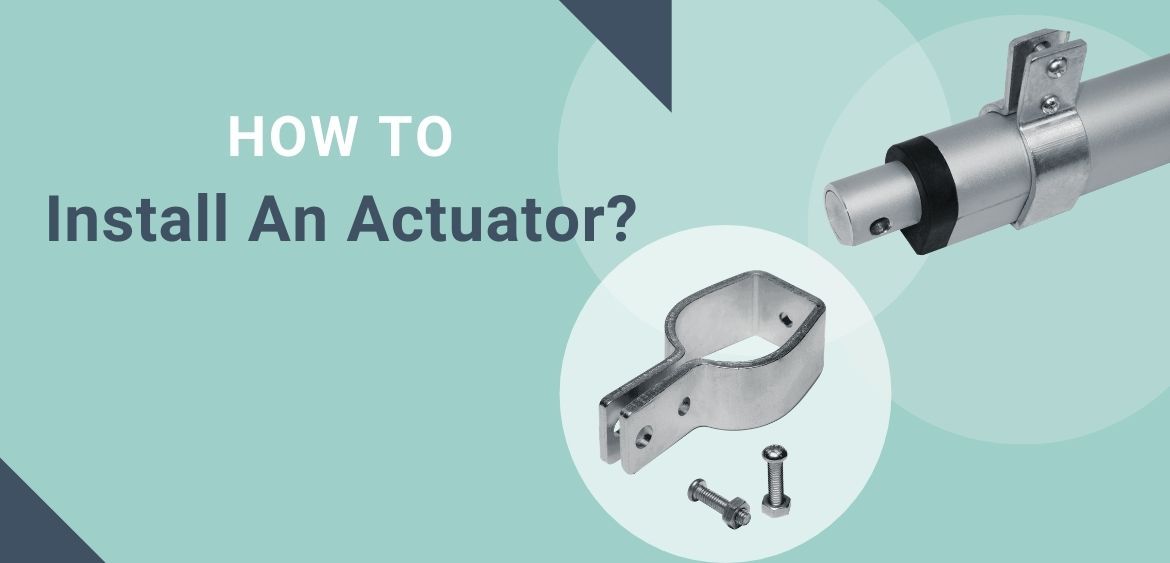The image serves as a header for an article on how to install an actuator, set against a turquoise background with a gradient pattern of white circles. The 'how-to' text appears in white on the left, followed by 'install an actuator' in blue. A prominent black triangle is positioned at the bottom left, while another oscillating black triangle extends from the top center. At the bottom of the image, there is a detailed illustration of a mechanical actuator with two screws and a large metal pole projecting from its right side, indicating where it will be connected. This setup is accompanied by a silver clamp with two adjacent Phillips head screws and a black plastic or rubber ring surrounding a smaller cylinder. The overall layout is accented by various shades of turquoise and gradient circles, enhancing the technical and instructional nature of the image.